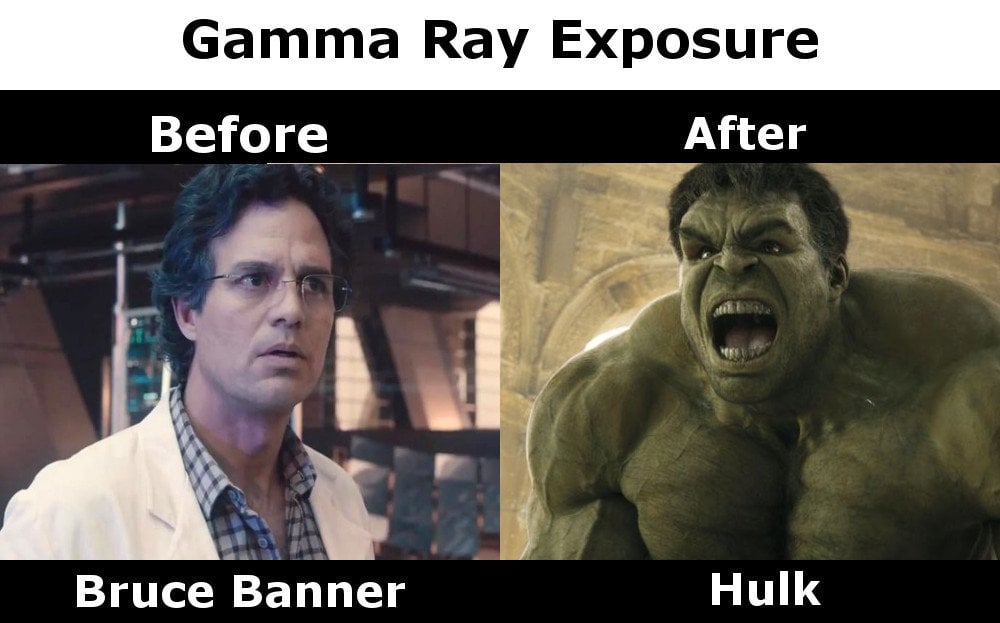The image is a meme format referencing the Marvel Comics character Bruce Banner and his transformed alter ego, the Hulk. It features two stills from Marvel movies positioned vertically next to each other. The top of the image has a white banner with black text reading "Gamma Ray Exposure." Above the left image, which depicts Mark Ruffalo as Bruce Banner, the text reads "BEFORE," and above the right image, which shows the Hulk in his transformed state, the text reads "AFTER." Bruce Banner is shown wearing a light cream jacket with a blue checkered shirt with white trim, round glasses, and has dark black hair, appearing puzzled in a lab setting. The Hulk, who is green with black hair, appears menacing with bulging muscles, an open mouth displaying green teeth, and an angry expression. The backgrounds indicate Bruce Banner is in a lab, while the Hulk is in front of a brick building. Underneath each image, there's a black bar with white text, stating "Bruce Banner" on the left and "Hulk" on the right.